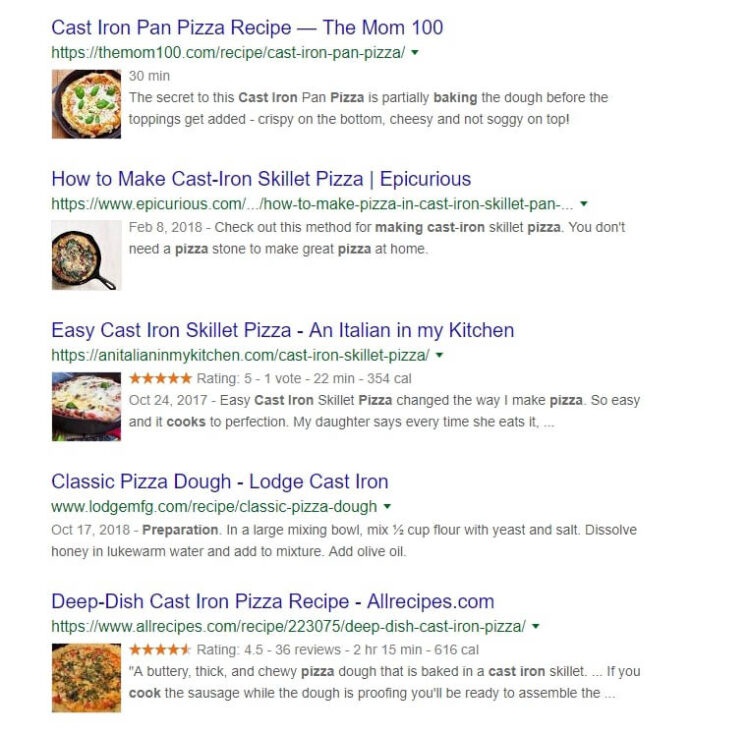This screenshot captures the top five Google search results for the query "cast iron skillet pizza recipe." The first listing is from Mom100.com, titled "Cast Iron Pan Pizza Recipe," indicating that the recipe takes 30 minutes to prepare. The second result, from Epicurious.com, is named "How to Make Cast Iron Skillet Pizza" and includes a brief content preview. The third link is "Easy Cast Iron Skillet Pizza from an Italian in My Kitchen" at AnItalianInMyKitchen.com, boasting a five-star rating and a 22-minute preparation time. Next is the "Classic Pizza Dough from Lodge Cast Iron," found on LodgeFMG.com. The final recipe, "Deep Dish Cast Iron Pizza Recipe" from Allrecipes.com, is rated 4.5 stars and has a preparation time of 2 hours and 15 minutes. Each listing provides a succinct preview of its content.